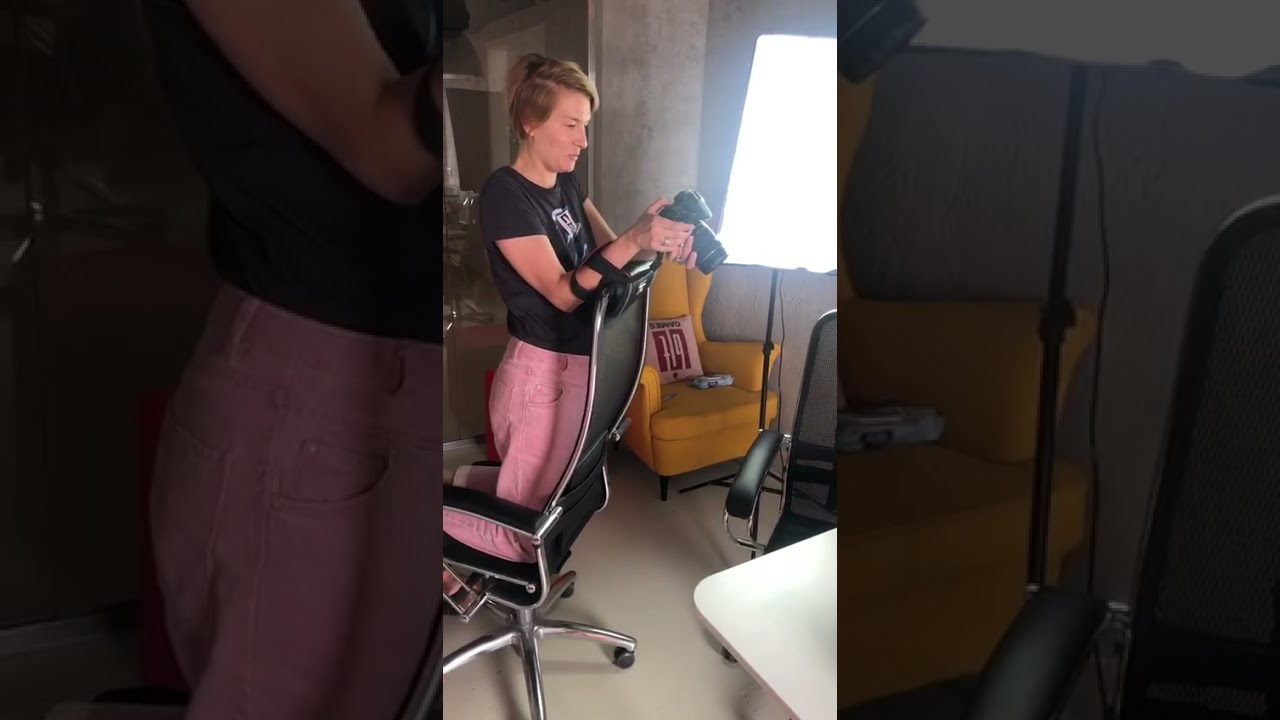This image is divided into three vertical sections, with the first and third sections featuring darkened close-ups of a central photograph. The middle section depicts a woman in a dimly lit room, kneeling on an office chair with wheels, her knees on the seat and her arms resting on the back of the chair. She holds a camera, seemingly taking a photo of something on a white table in front of her. The woman is dressed in a black t-shirt and pink pants. Positioned to the left of the woman is a yellow armchair with a pink and red throw pillow. The black office chair she kneels on has a silver metallic boundary. The room's floor is made of white tiles, and the walls are gray. A bright white light shines into the room, enhancing the overall darkened ambiance. In the right section, another black office chair and the white table are visible near a window that casts the illuminating light. The scene captures the woman engrossed in her photography, with a professional camera pointing downward over the chair’s back, possibly towards the table below.